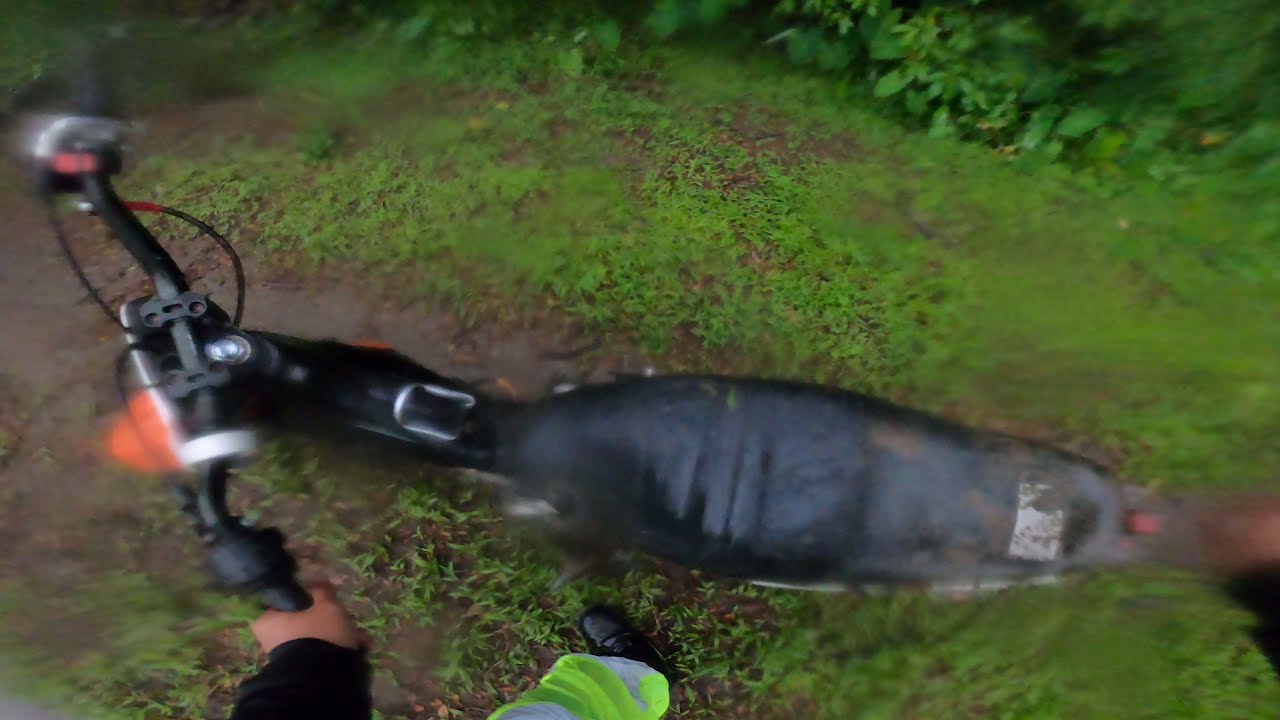This photograph, taken from above, captures a black motorbike resting on a muddy and grassy terrain. The bike features a black seat and black, white, and orange handlebars adorned with brake cables. The ground beneath is wet and muddy, with patches of green grass interspersed. To the side, some low green vegetation and larger brushy plants are visible, hinting at the edge of a woodland area. The person partially visible in the image wears lime green pants and black shoes, with one hand gripping the left handlebar of the bike. The photograph is slightly blurred, emphasizing the rugged, damp environment surrounding the motorbike.